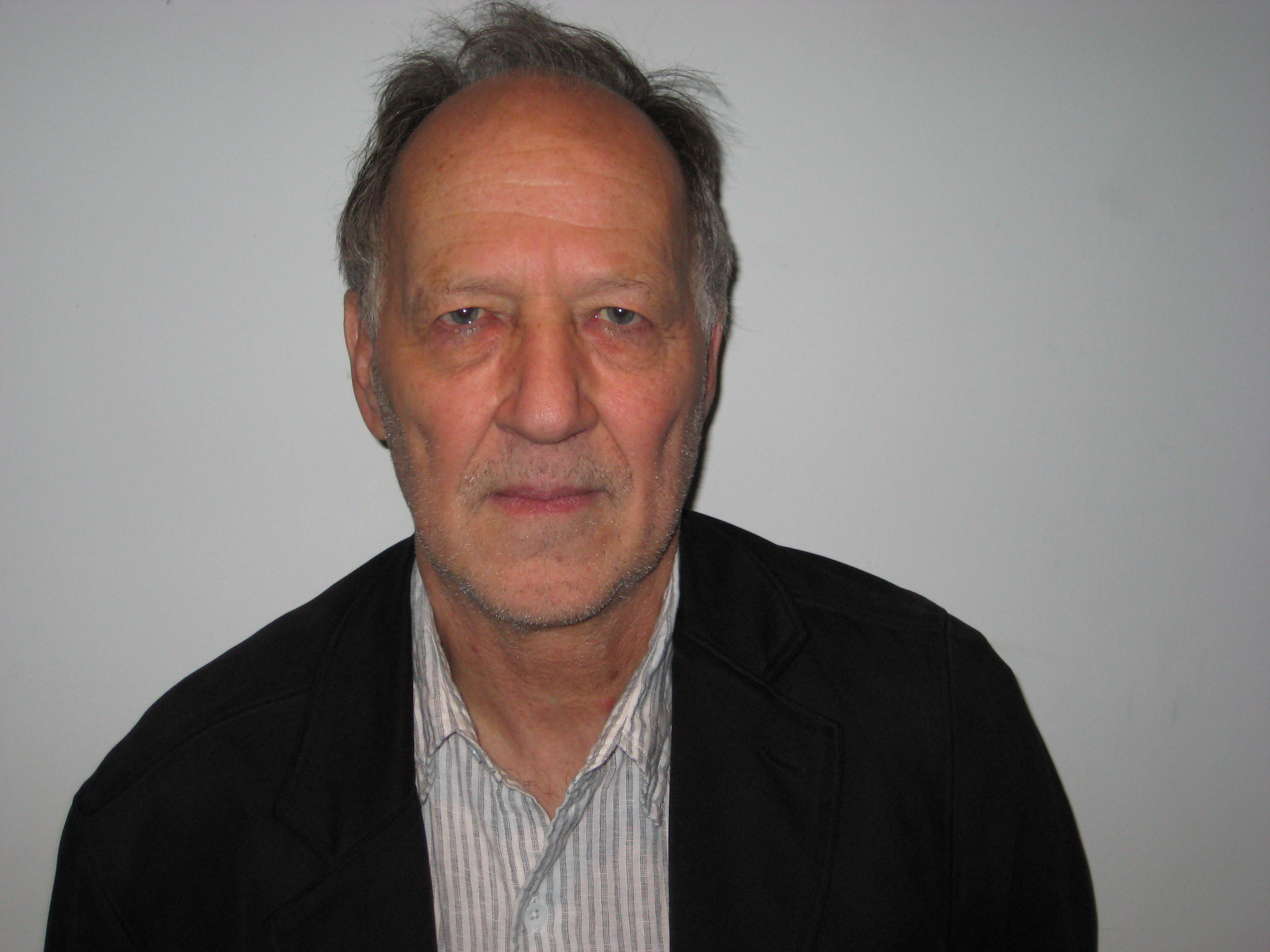This is a photograph of actor, director, screenwriter, and producer Werner Herzog, an older white male with a receding hairline and disheveled dark hair streaked with gray. He is slightly unshaven, adding to his rugged appearance, and has droopy eyelids with heavy bags under his eyes, contributing to a weary yet intense expression. Herzog is wearing a white and gray striped collared button-down shirt underneath a dark sweater or light jacket with an open front. He is seated against a background that appears to be either white or a varying shade of gray, staring straight into the camera with a serious demeanor. The image captures Herzog's distinguished yet solemn presence.